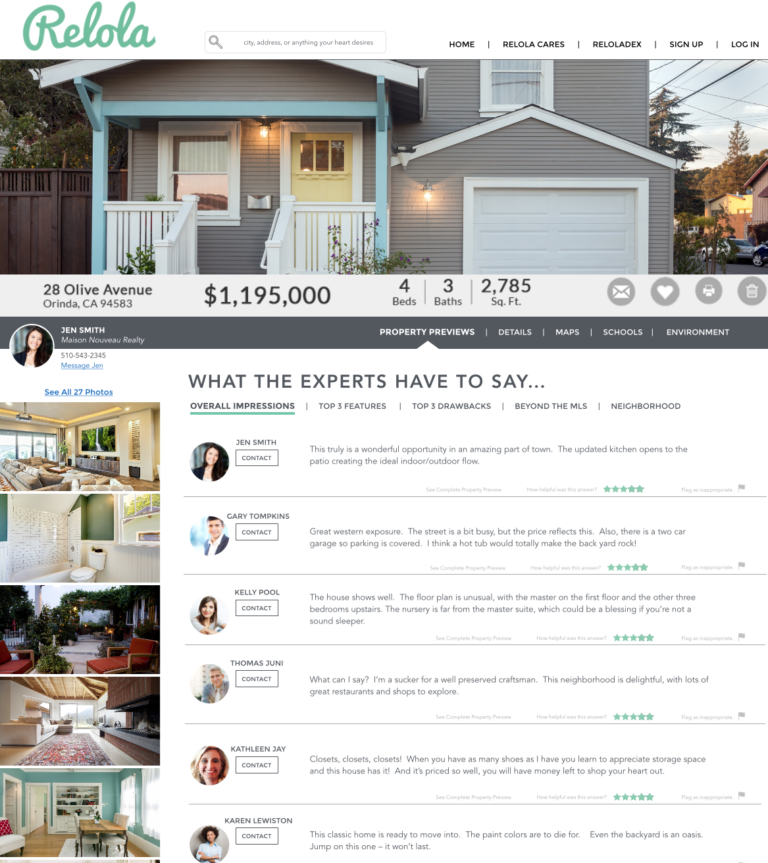Screenshot of RELOLA Webpage Featuring a Detailed House Listing

At the top of this RELOLA webpage, the RELOLA logo is prominently displayed in the upper left-hand corner. The page is visually dynamic, filled with various pictures of a house and its interior. This webpage serves as a comprehensive listing for a house currently for sale.

Top Navigation and Search Features:
- A search bar sits at the very top, allowing users to search for a city, address, or anything else they desire.
- Next to the search bar, the navigation menu includes options for "Home," "RELOLA Cares," "RELOLA Decks," "Sign Up," and "Log In."

Main Listing Information:
- The featured image is an exterior photo of a single-family home with a garage and a porch. The house is gray in color.
- Address: 28 Olive Avenue, Orinda, California 94583.
- Price: $1,195,000.
- Details: 4 bedrooms, 3 bathrooms, and a total living space of 2,785 square feet.
- Additional interactive icons include options to email, favorite (heart icon), print, and delete (trash can icon).

Realtor Information:
- Displayed on a wide, gray bar across the page's width, the realtor information is clearly laid out.
- Realtor: Jen Smith from Maison Nouveau Realty.
- Contact: Phone number 510-543-2345 and an option to message her directly.
- A circular photo of Jen Smith is next to her contact details.
- Menu options on this bar include "Property Previews," "Details," "Maps," "Schools," and "Environment," with "Property Previews" currently selected.

Expert Opinions and Ratings:
- Section titled "What the Experts Have to Say" allows visitors to read expert reviews.
- Sub-sections include "Overall Impressions," "Top Three Features," "Top Three Drawbacks," "Beyond the MLS," and "Neighborhood," with "Overall Impressions" currently selected.
- Several quotes with five-star ratings from different realtors or experts provide insights and reviews about the house. Contact buttons are available for each reviewer.

Photo Gallery:
- On the left-hand side, a vertical listing of interior photos is displayed.
- Visitors can see images of the living room, bathroom, outdoor patio, and dining room, with an option to "see all 27 photos" for a more detailed view.

This detailed caption showcases the comprehensive and user-friendly layout of the RELOLA webpage, providing prospective buyers with all necessary information and convenient navigation tools to explore the house listing further.